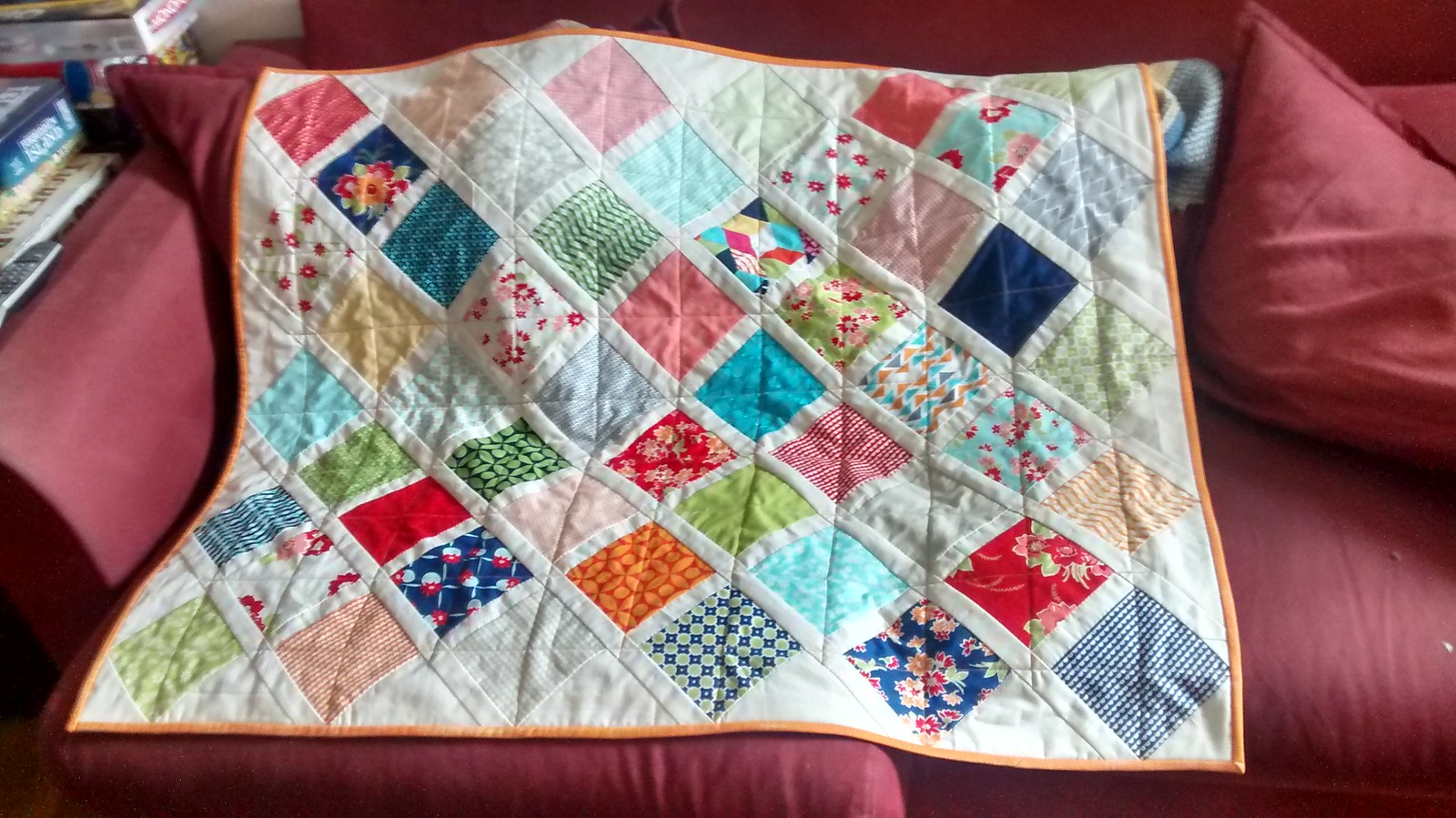The photograph showcases a handmade patchwork quilt laid out across a wine-colored sofa, offering a full view of the intricate design. The quilt is composed of multiple rows of squares, each featuring a unique patchwork pattern of various cloth materials. The background color is a pristine white, complemented by fairly thick crisscross lines that create distinct borders for each square. These lines are also white, adding a subtle yet cohesive contrast to the colorful patches. The quilt is framed by an orange border, providing a vibrant edge to the overall design. In the background, to one side of the sofa, there is a small stack of books and a plastic container, likely filled with sewing supplies. The scene is softly illuminated by natural ambient light, enhancing the quilt's details and the cozy setting. No text is present in the image.